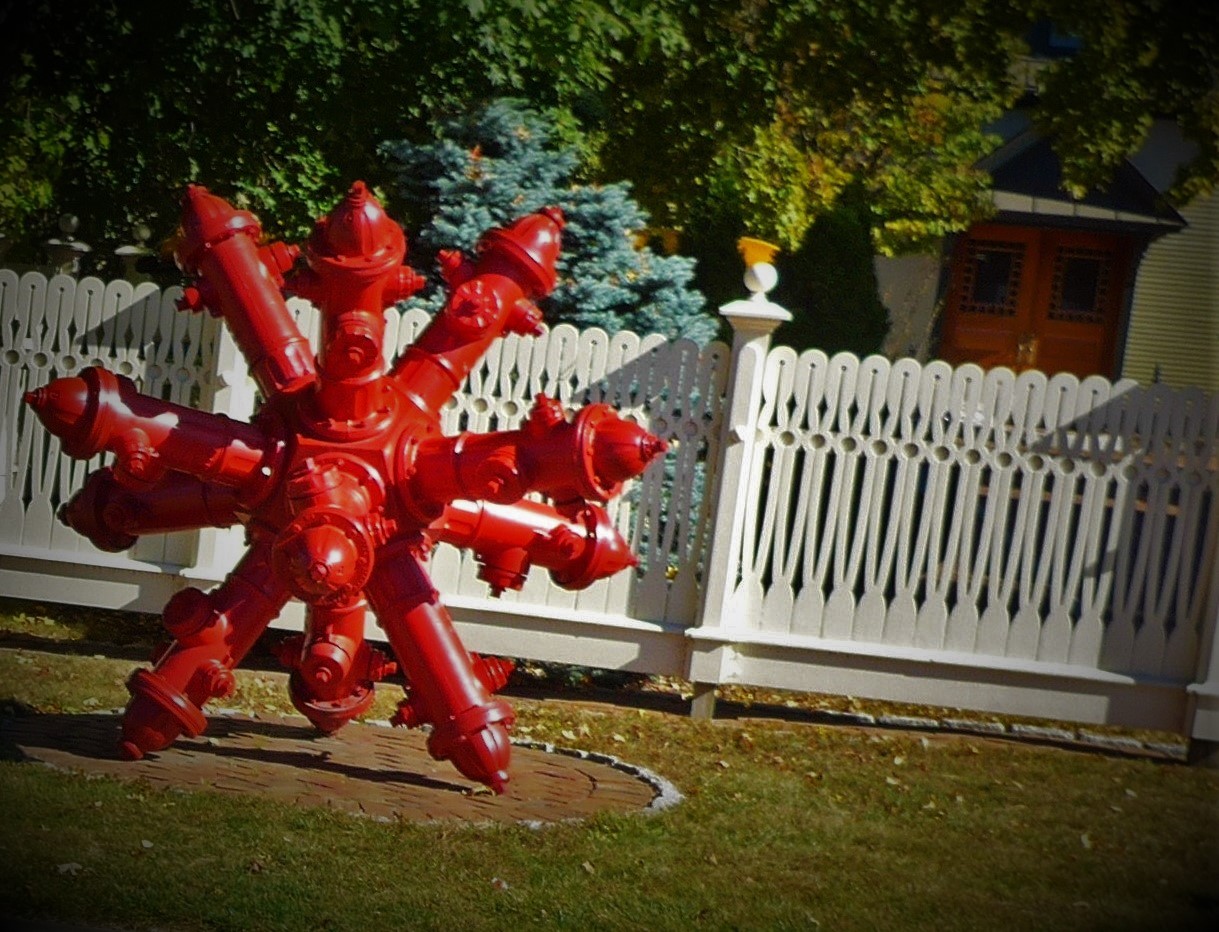The image portrays a detailed outdoor scene, featuring a house with two wooden doors set in the background. This house is partially obscured by a white, vinyl fence, reminiscent of a picket fence but with an intricate design. Surrounding the area are various trees, including a vibrant green one and an evergreen. In the foreground, there is a grassy hill peppered with a few scattered leaves. Centrally located on the grass is a round section bordered by bricks and rocks, containing an unusual and striking red statue. This artwork is designed to resemble a giant version of a jack from the children's game but is composed entirely of multiple fire hydrants. Each hydrant radiates outward from a central sphere, creating a visually arresting sculpture that stands out against the natural setting.